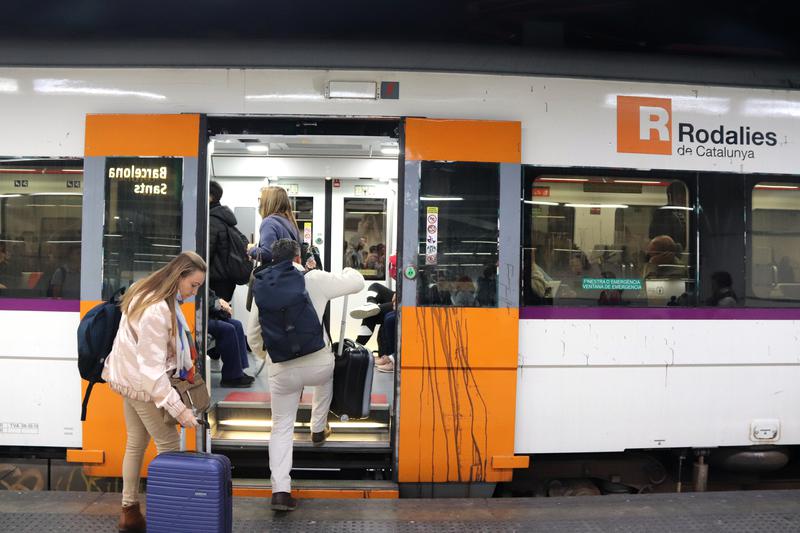In a bustling subway station, a sleek white train adorned with purple trim beneath its windows and the logo of an orange square with a white "R" alongside the text "Rodalies de Catalunya" pulls into view. The train features striking orange and grey doors, which stand open, ready for boarding. At the forefront, a man dressed entirely in white, wielding a blue backpack and a black roller bag, steps confidently onto the train. His short black hair contrasts sharply with his outfit. Directly behind him, a woman with long light brown hair, clad in a white jacket with fringe, tan trousers, and hiking boots, waits her turn to board. She balances a black backpack over one shoulder and steadies a blue suitcase with her other hand, poised to follow him into the train. The scene captures the daily commute with a vibrant palette and the quiet choreography of passengers in motion.